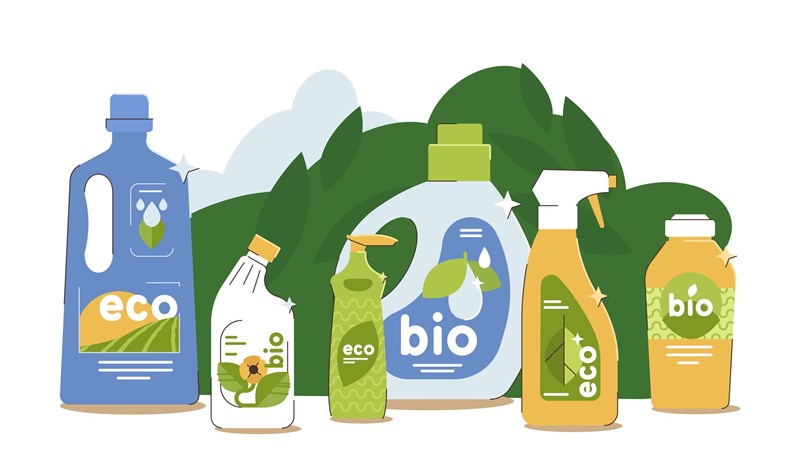This artist's illustration showcases a variety of environmentally friendly cleaning products, depicted in an abstract, animated style. The lineup includes six different items: a blue-handled container labeled "eco," presumably a detergent; a white bottle with the word "biome," possibly a toilet cleaner, adorned with an image of a sunflower; a green pump container labeled "eco," likely hand soap or dish soap, accented by a dark green leaf; a primarily blue laundry detergent bottle featuring the word "bio" and a shiny water drop; a yellow-background spray bottle tagged "eco," suggesting a multi-purpose cleaner; and another yellow-background bottle labeled "bio," its exact use unclear, perhaps hand lotion or dishwasher detergent. The background is filled with abstract green leaves and bushes, reinforcing the eco-friendly theme. The overall color scheme includes dark green, blue, and orange, with muted tones, emphasizing the natural and organic nature of the products.